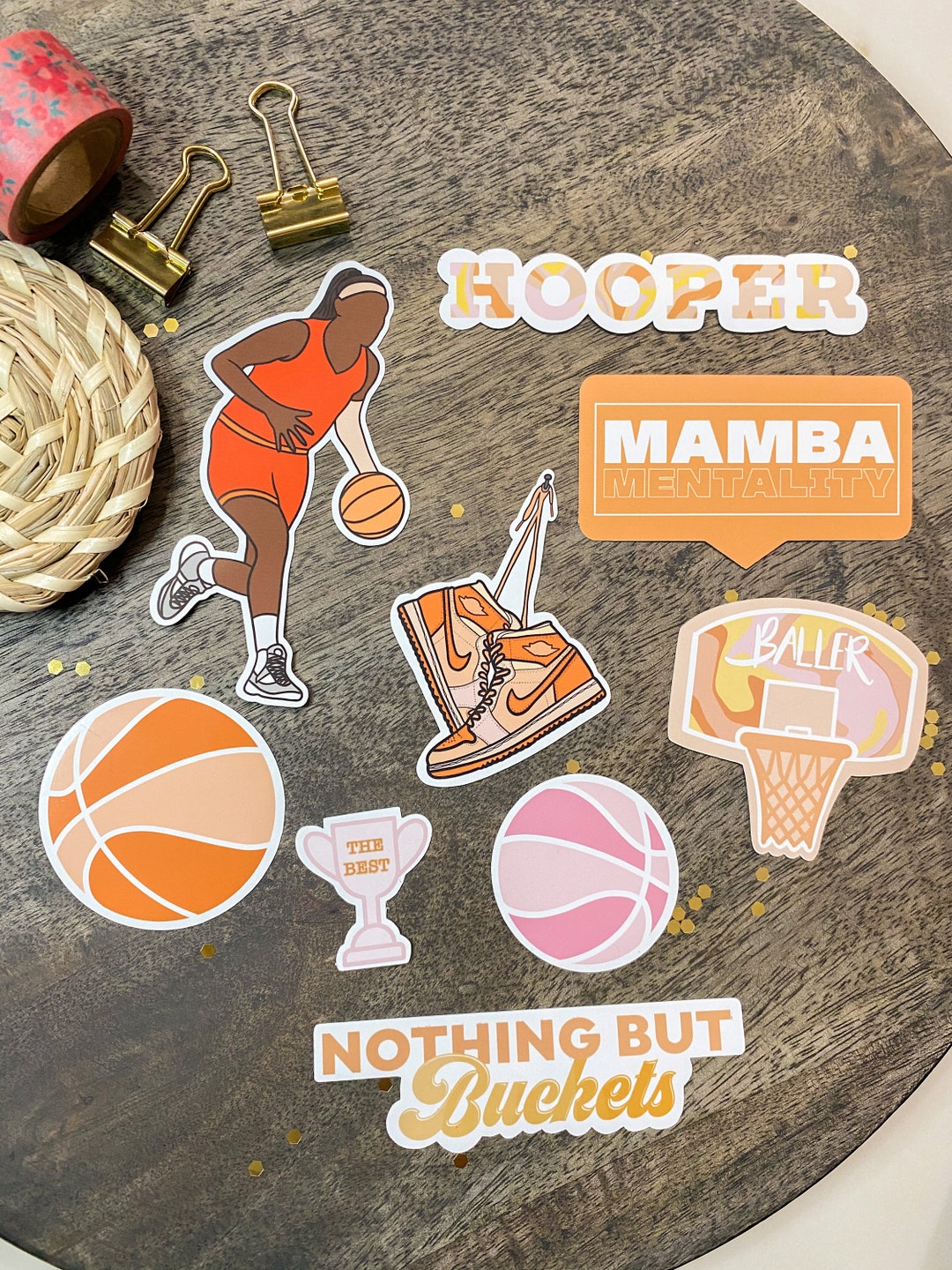The image features a circular, dark wooden plate adorned with various stickers and decals. At the top right is a sticker that reads "Hooper" in mixed orange and yellow hues with a white outline. Below it, a large rectangular speech bubble in orange contains the bold white text "Mamba" and underneath it "mentality" in white outline with an orange fill. There is also a sticker of a basketball hoop with the word "baller" across the backboard, which has hues of yellow and orange.

To the left of the "Hooper" sticker is an illustration of a female basketball player with dark skin, wearing a red jersey and shorts, dribbling a basketball. To the right of the "Hooper" sticker is a pair of orange and light orange Nike sneakers attached by a pin through the shoelaces. Below it sits a pink basketball.

Further down, a trophy sticker to the left reads "The Best" while adjacent to it is an orange basketball. Another sticker below the pink basketball and the trophy says "Nothing but buckets" in bold text. The placement of these vibrant stickers creates a dynamic and energetic collage, radiating themes of basketball and athletic spirit.